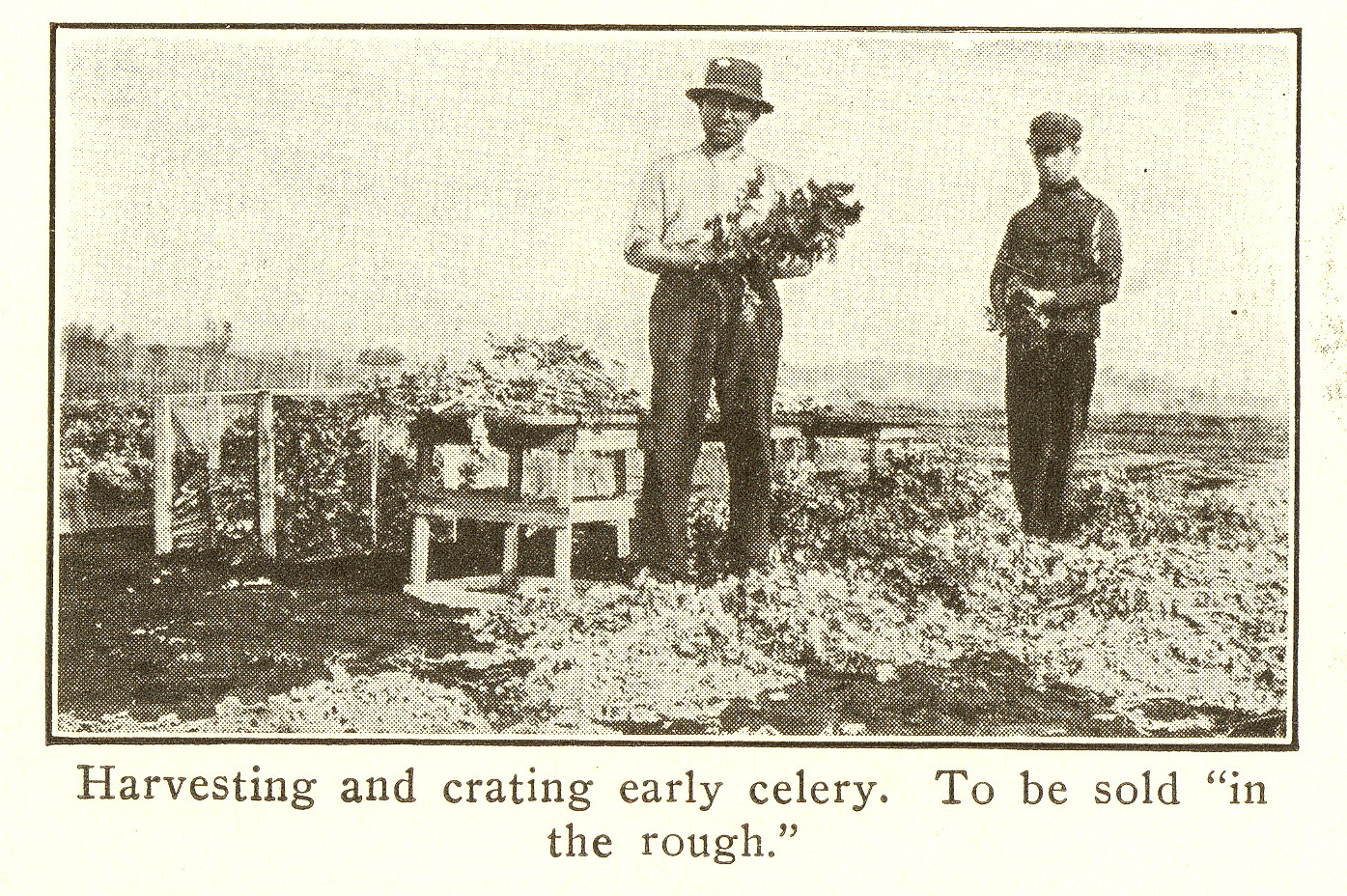This grainy black-and-white photograph, tinged with a cream-colored tone, features an old and smudgy print capturing a rustic farmland scene. At the center stands a man clad in a light-colored plaid button-up shirt, black pants, and a bucket hat, holding leafy vegetables in both hands. Next to him, on the right, is another man wearing a cap, a dark plaid shirt, and black pants, also holding some leafy crops. The background shows a plain with visible dirt in the bottom left corner, presumably mountain dirt, and hints of some crops, possible fencing, and crates, though the image's low quality makes it difficult to discern details precisely. A table near the central man displays an array of crops, presumably vegetables. The backdrop fades into a grainy, cloudless skyline. Below the image is a caption bordered in black on a white background, reading: "harvesting and creating early celery to be sold (in the rough)."